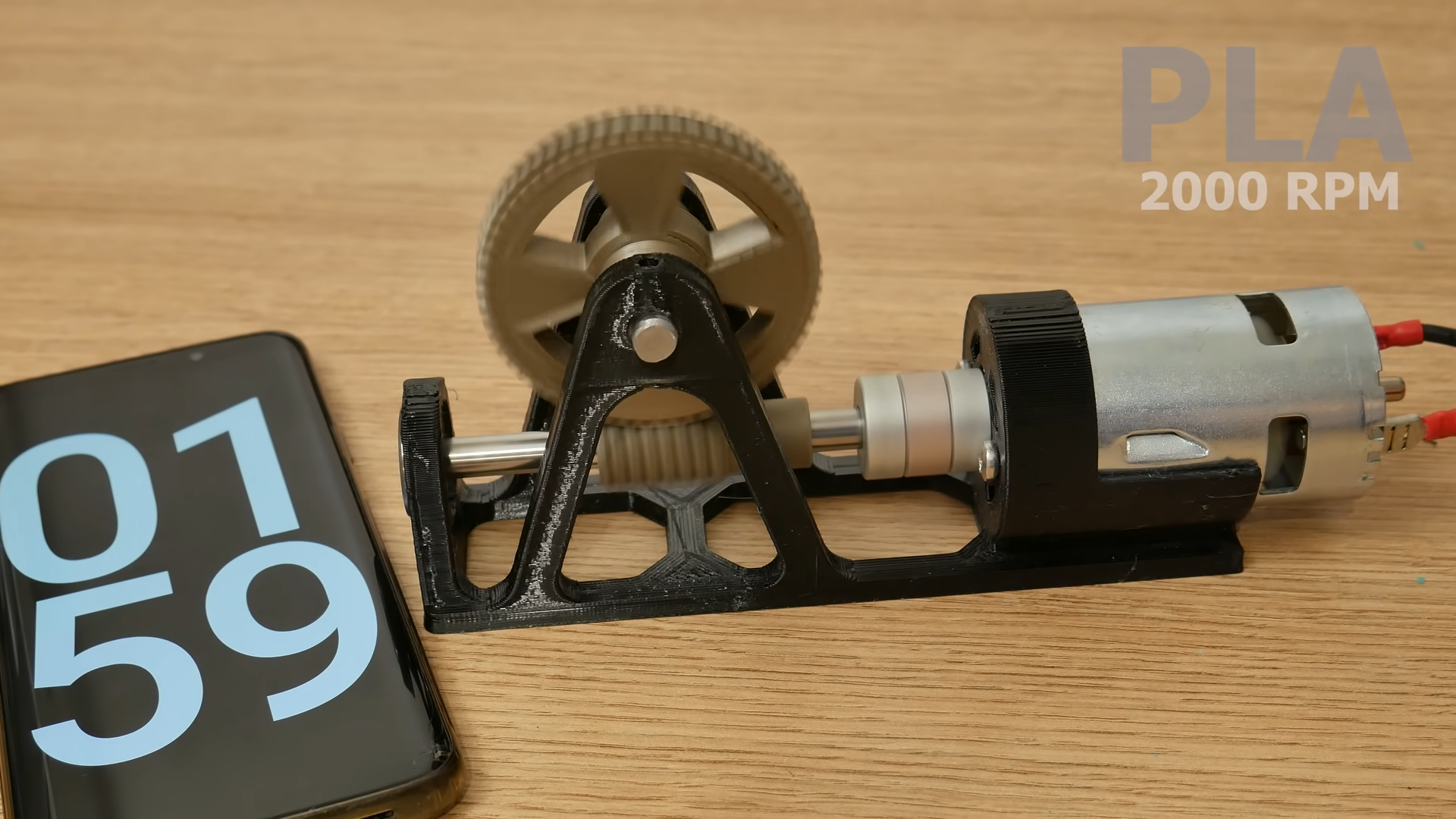This photograph captures a close-up of a compact, handmade 3D-printed device positioned on a wooden table against a black background. To the right, there are several wires equipped with clamps and red plastic protectors, which are attached to a large silver cylinder. This cylinder appears to be part of a motor assembly featuring a brownish, grooved plastic cylinder within it and what could potentially be magnets at the end. There is also a noticeable gold-colored wheel that spins beside the motor. 

Nearby, a small black tile or label displays the numbers "0159" with "0" and "5" on the top row and "1" and "9" on the bottom row. The black frame of the device, which has a cast iron appearance but is actually 3D-printed, somewhat resembles a flat bicycle frame. Adjacent to this assembly, there is a cell phone, suggesting that the entire setup is relatively small. The words "PLA 2000 RPM" are visible in the upper right corner, further indicating the device's operational speed. Overall, the assembly appears to be a scientific or experimental contraption, quite possibly a small motor or a tool.